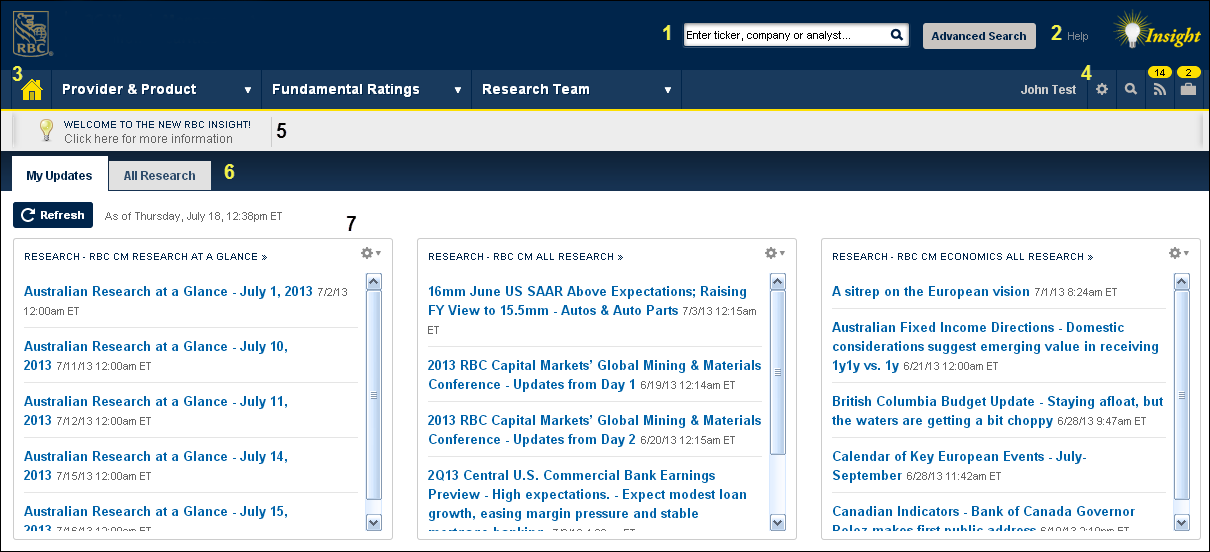In the top left corner of the image, the RBC logo is prominently displayed, while the top right corner features the Insight logo accompanied by a light bulb icon. Below these logos, there is a search bar designed to enter a ticket, company, or analyst for advanced search purposes. 

Directly underneath the search bar is a navigation bar with multiple options: "Provider and Product," "Fundamental Rating," and "Research Team," each with its own drop-down menu. Beneath the navigation bar is a welcoming message that reads, "Welcome to the new RBC Insight, click here for more information."

Further down, the page offers two options: "My Updates" and "All Research," with the current page being "My Updates." This section includes a "Refresh" option. Below this, there are several entries titled "Australian Research at a Glance," each dated respectively: July 1st, 2013, July 10th, 2013, July 11th, 2013, July 14th, 2013, and July 15th, 2013.

In the middle column, a headline reads, "16mm June US SSAR above expectations raising FY viewed to 15.5mm autos and auto parts." In this section, there are also four additional clickable links. Adjacent to this column is another section featuring five different clickable links, each directing to various research documents.